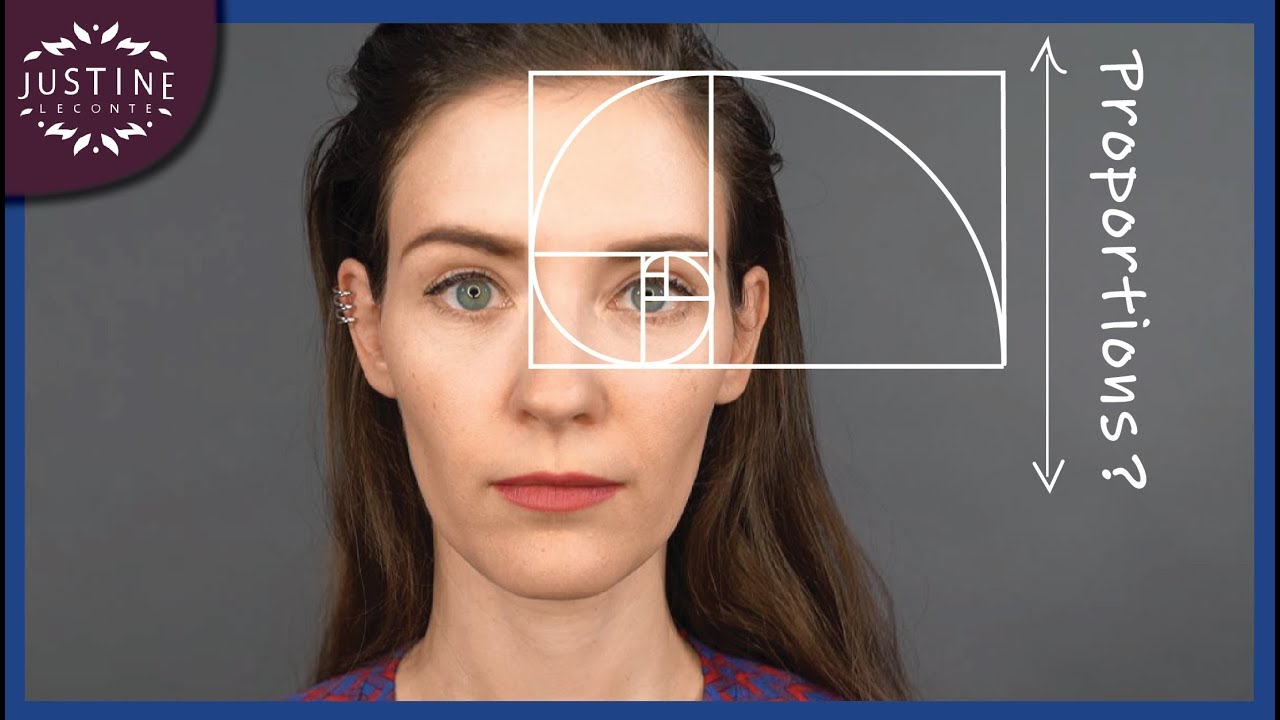The image is an instructional photograph with various overlaying designs and text. It features a woman facing the camera with her eyes wide open and mouth closed. She has long, somewhat wavy brown hair that's pulled up at the front and flows in the back. Her bluish-green eyes are accentuated with eyeliner, and she is wearing medium red lipstick. In her right ear, she has three silver cartilage hoop earrings. 

A distinctive golden spiral diagram overlays her left eye, suggesting an ideal proportionality. The spiral, contained within a white rectangular box, begins at her eye and expands outward, with several lines emanating from it. To the right of this diagram, an arrow with arrowheads points up and down, accompanied by the word "proportions" followed by a question mark.

The photograph itself has a gray background and is bordered by a blue frame. In the top left corner of the image, there is a logo featuring ornate design elements and the name "Justine Leconte" written in white within a purple space with rounded edges. The overall composition seems to emphasize the symmetrical and proportional aspects of her face using the golden spiral diagram.